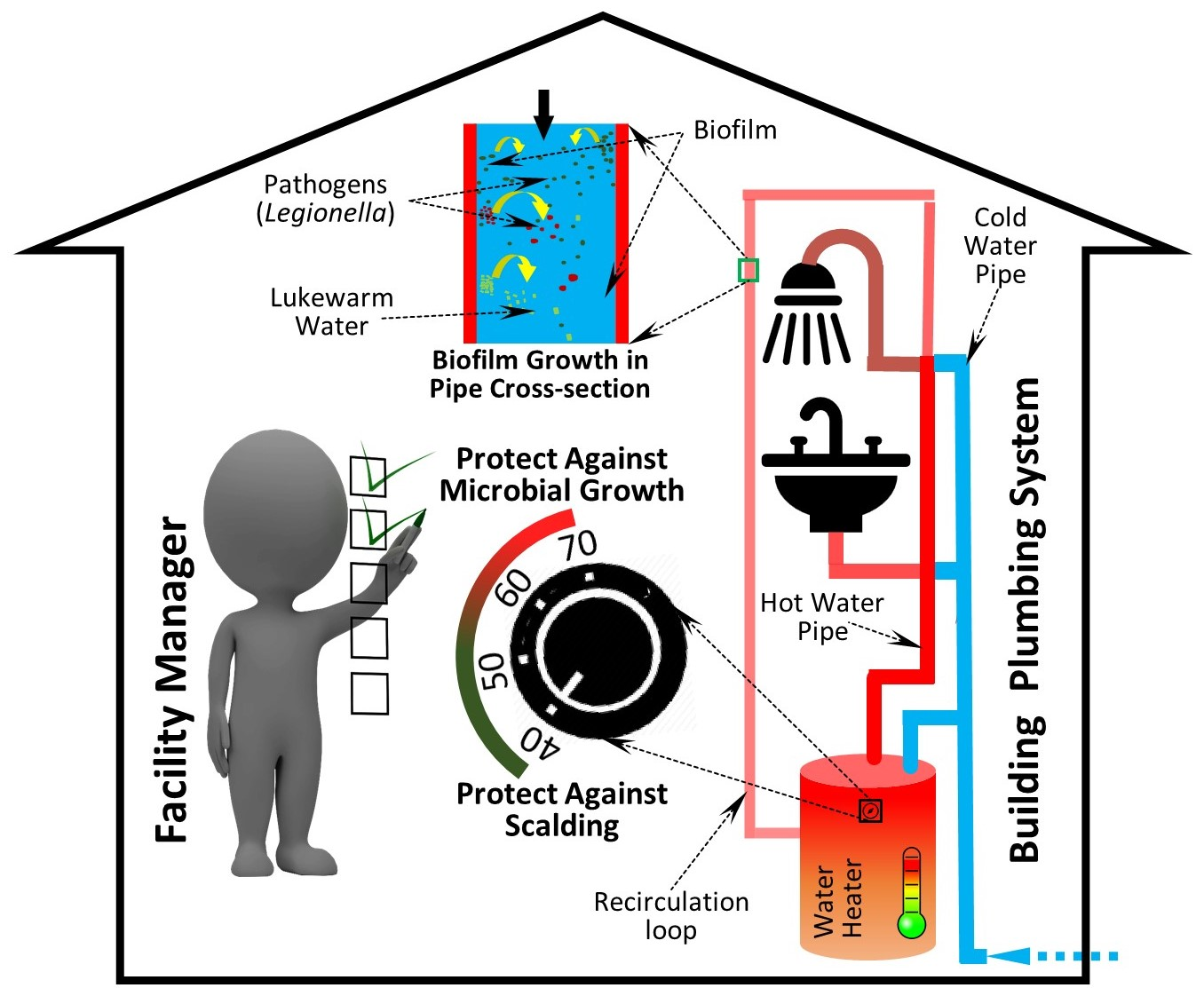This detailed diagram of a house illustrates the proliferation of microbes within its plumbing system. The black outline of the house frames various illustrated components: a L-shaped water heater with incoming cold water and outgoing hot water pipes, leading to fixtures like a sink and shower. Vertical text on the left side identifies the Facility Manager, depicted as a simplistic gray stick figure without facial features, pointing at a section marked "Protect Against Microbial Growth" with only two out of five checkboxes ticked.

On the right side, another vertical label reads "Building Plumbing System," highlighting the water heater, hot and cold water pipes, and a recirculation loop. The diagram emphasizes microbial hazards such as biofilm, pathogens, and Legionella, indicated particularly within lukewarm water sections. Temperature regulation, crucial for microbial control and scald protection, is represented by a temperature dial ranging from 40 to 70 degrees Celsius, with emphasis on setting it correctly to mitigate both microbial growth and scalding risks. The detailed layout blends these components into a comprehensive visual explanation of potential microbial growth zones and maintenance points within a household plumbing system.